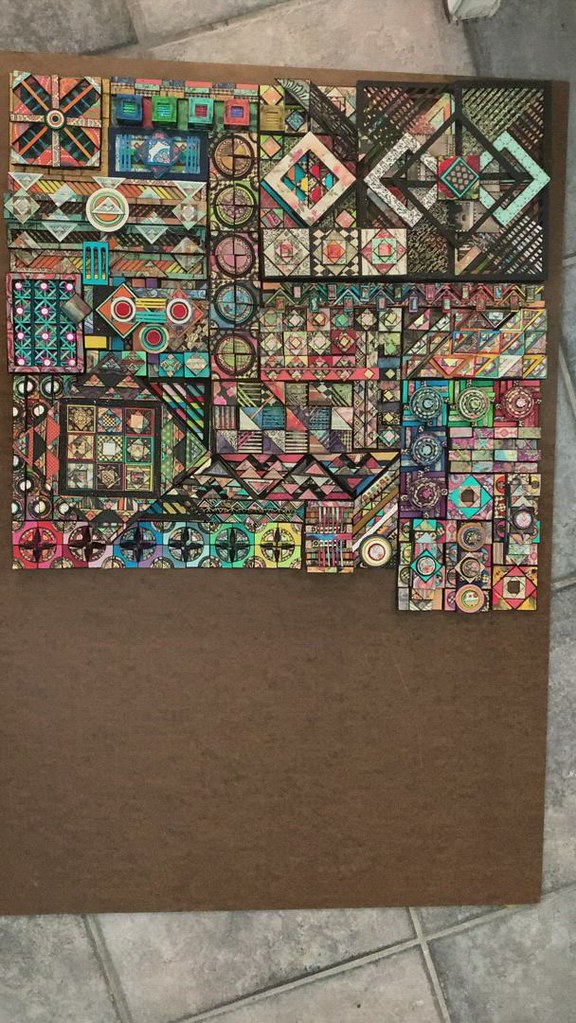The image showcases an intricately designed floor with various elements. The base comprises stone tiles meticulously arranged on the ground. At the center lies a large, square piece framed by these tiles, featuring a rich brown felt texture. This central square is an artistic mosaic made up of different ceramic tiles, each showcasing unique patterns and colors.

In the top left section, there is a black cross accented with red and white designs. The mosaic radiates a vibrant blend of hues including blue, green, white, red, pink, and yellow, forming circles, diamonds, crisscross patterns, and deformed checkered motifs. The array of shapes continues with triangular, cross-like, and additional geometric designs, contributing to the overall impression of a diverse and creative tile composition, reminiscent of a tapestry of artistic expressions.